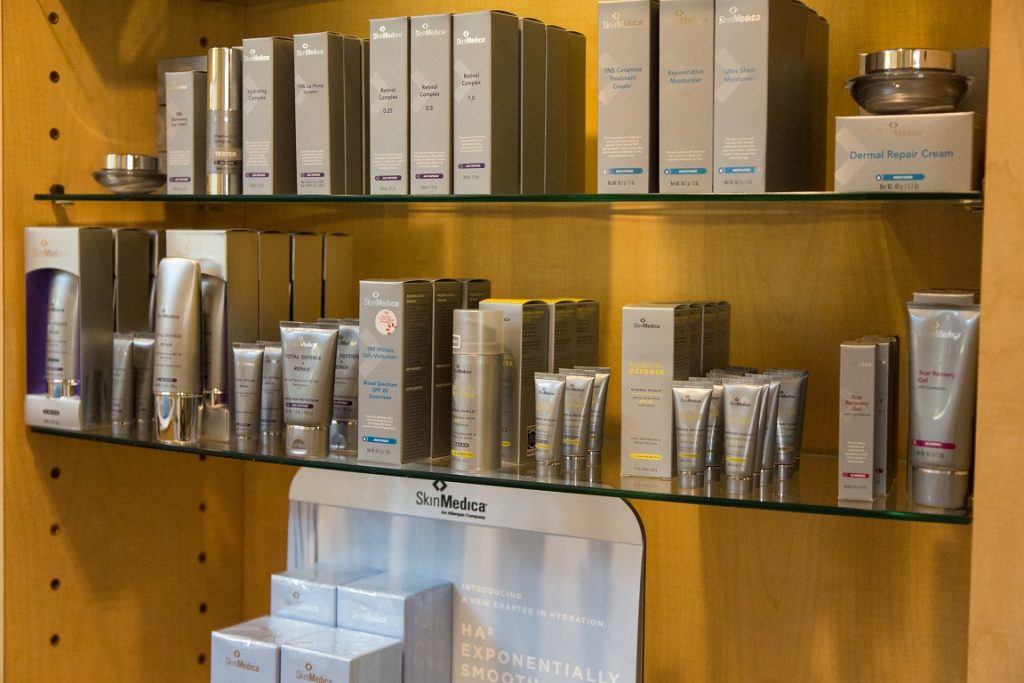The image depicts a high-end skincare display set into a wooden cabinet with a camel brown finish. The cabinet features two glass shelves and an obscured bottom shelf. On the top shelf, there are nine mauve-colored boxes with shiny, engraved writing and small color bars at the bottom, standing in an organized manner. The three boxes at the center and right are closely packed together, while the leftmost three have a bit of space between them. Positioned between the leftmost and second boxes is a gold cylindrical jar, possibly a makeup cream bottle, with another larger jar placed on top of a box to the right. Below, on the second shelf, a matching color scheme is maintained with an assortment of shiny, sandy gray and beige tubes of various sizes—small, medium, and large—neatly lined up alongside the boxes. The bottom part of the display showcases a white background with four more light gray or whitish boxes arranged in two rows, with the taller ones behind. The entire elegant setup hints at premium skincare products, with a product labeled "Dermal Repair Cream" and a display that reads "Sun Medica" at the back.